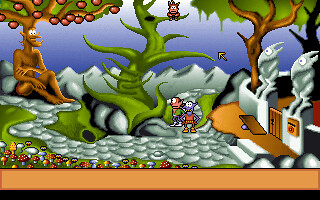Caption: 
A nostalgic screenshot from an old-school, two-dimensional, low-resolution, side-scrolling video game capturing an outdoor scene. A gray stone path winds through lush green grass, flanked by a variety of intriguing trees. One tree features a carved trunk resembling a monkey and bears fruit in its branches, while another resembles a tangle of large green vines, upon which a small creature perches. In the background, a sturdy gate and adjacent wall host two imposing, gray statues with alien-like features. In the center of the screen, two alien-looking creatures stand, possibly engaged in an interstellar dialogue. The bottom left corner of the image showcases a dense cluster of mushrooms or other small flora, adding to the scene’s intricate and whimsical charm.